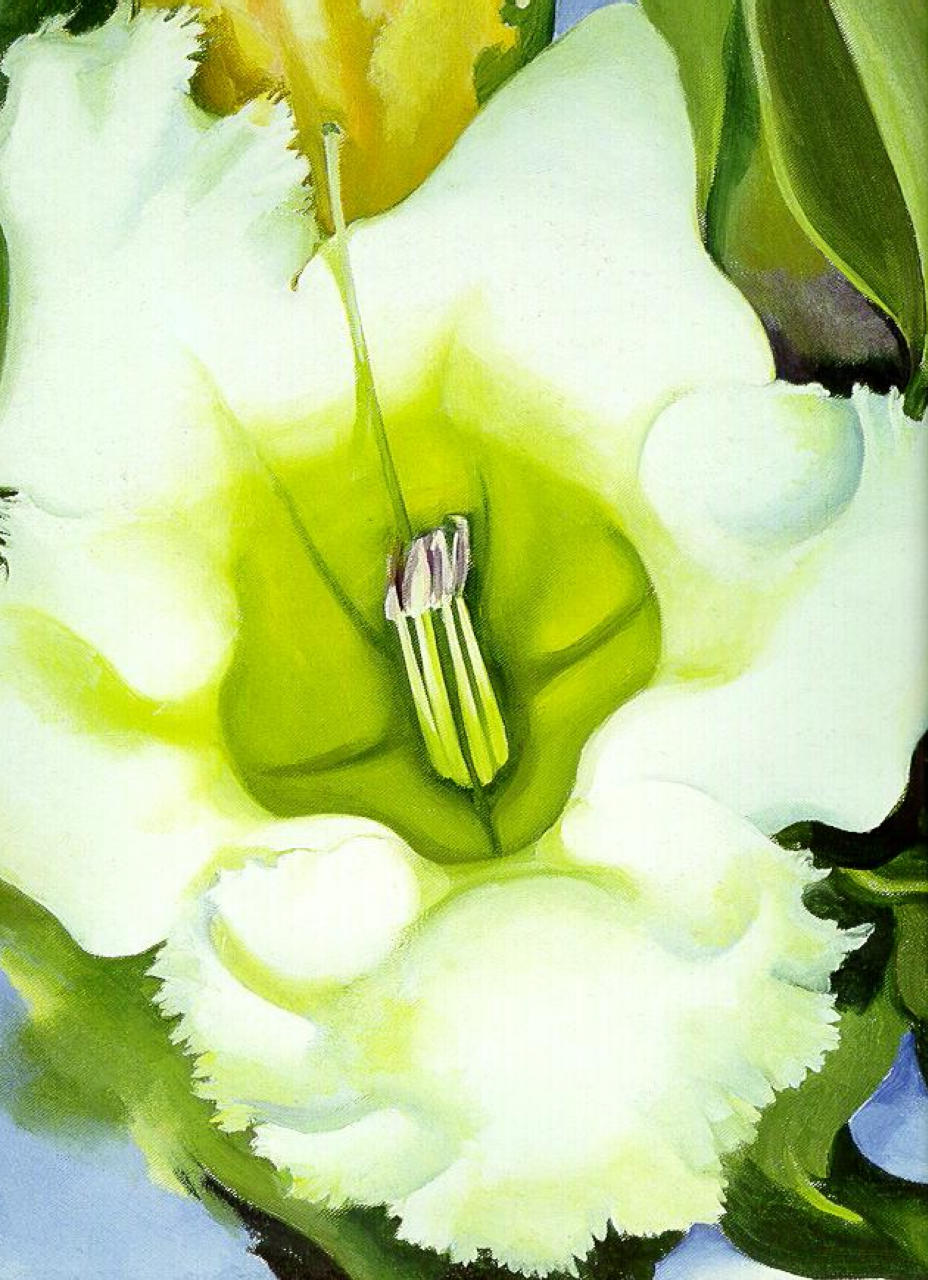This painting, possibly rendered in watercolor or oil paint, captures a close-up view of a flower's intricate interior. Dominating the composition is a cream-colored flower that transitions to a vibrant green at its center. Its four petals, which are triangular at the tips and rounded at the base, feature a ragged, fringed border with light green and yellow accents. The detailed center of the flower showcases rod-like stamens and pistils that are green at the base and transition to a mix of purple and white at their tips. Surrounding this central bloom, the painting includes a vibrant yellow flower in the background, as well as wavy green leaves that encircle the scene, appearing both at the bottom and top right corner. Hints of blue at the lower left and right corners, and subtly at the top, suggest the presence of the sky and add depth to the overall composition. The painting is rich in color and finely detailed, with no text to distract from its natural beauty.